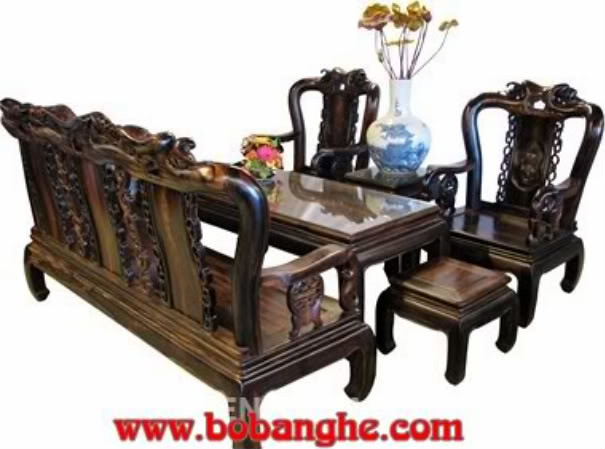The image appears to be a photograph, likely from an advertisement, showcasing an ornately designed dining set made of highly polished, solid wood. At the center is a long, shiny wooden table with intricate carvings and traditional Asian motifs, including dragon figures and lucky coin designs. One side of the table features a beautifully carved wooden bench, while the other side has two smaller, heavily carved chairs with bow-legged bases and dragon motifs. Additionally, there's a small matching step stool and a side table situated between the two chairs, topped with a Ming-style white vase adorned with blue and gold flowers, likely artificial. The overall set exudes a regal and antique charm, suggesting high-quality craftsmanship. The furniture has a waxed sheen, indicating careful maintenance. At the bottom of the image, there is a red text reading "www.bobanghe.com," in an artsy font, partially obscured by a white watermark showing the letters "E" and "N."